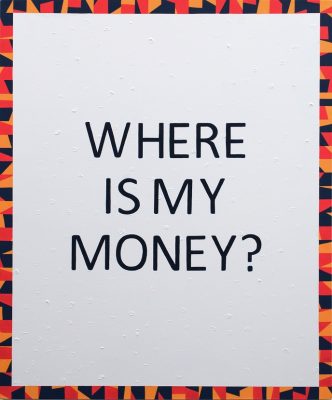This image is a vertically formatted rectangular poster with a prominent message in uppercase black letters reading, "WHERE IS MY MONEY?" The text is centered on a plain light gray (or white) background. The message is displayed across three lines, with "WHERE" at the top, followed by "IS MY" in the middle, and "MONEY?" at the bottom. Surrounding this central text is a colorful border featuring an abstract geometric design. The border incorporates jagged and stained-glass-like shapes primarily in red, yellow, dark blue (almost black), orange, and pink. The overall aesthetic is striking due to the contrast between the simple text and the vibrant, patterned border.